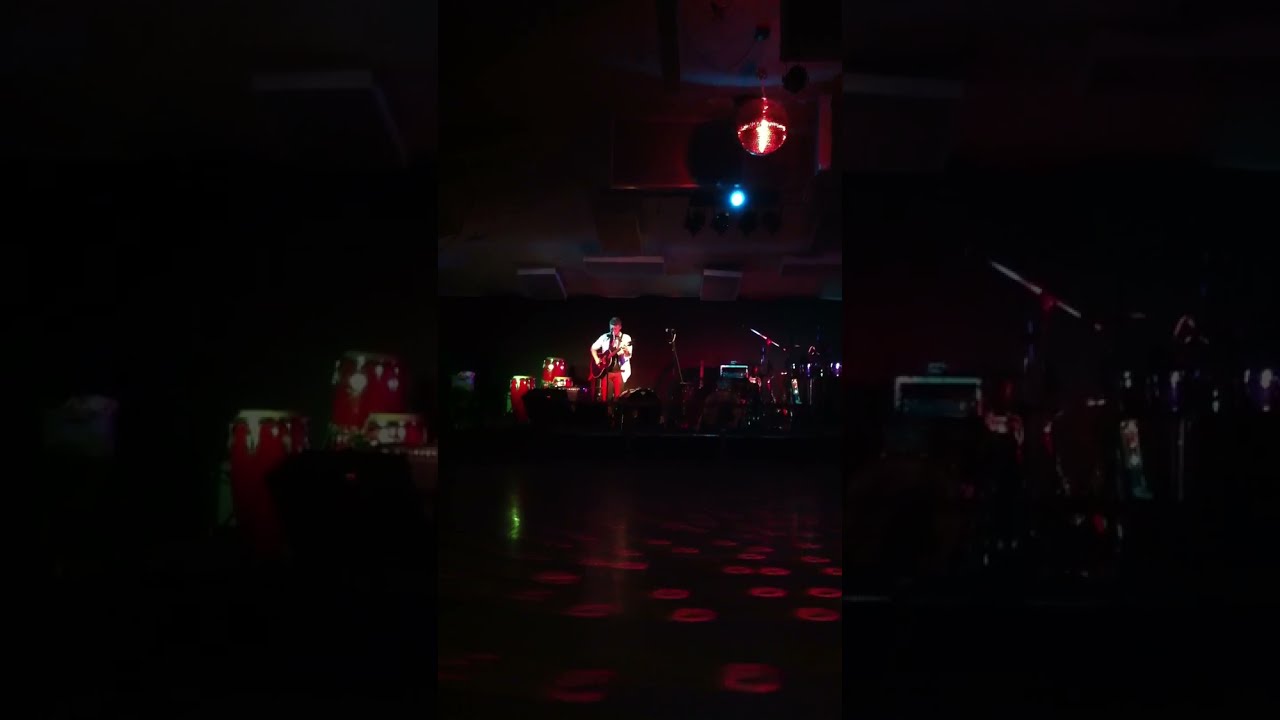In a dimly lit room, a musician commands the stage, surrounded by a scattering of musical instruments. The foreground reveals an empty dance floor, marked by numerous footprints and illuminated by neon green and red reflections from ceiling lights. A glittering disco ball hangs in the top right, casting an orange and red glow across the scene. The performer, a man with possibly spiky blonde hair, stands before the leftmost of three microphones. He wears striking red pants and a long white jacket, skillfully playing an acoustic guitar while singing. Behind him, a set of drums and other musical equipment are faintly visible under the subdued stage lighting. Overhead, the ceiling is adorned with ductwork and air vents, barely discernible in the darkness that envelops the rest of the venue.